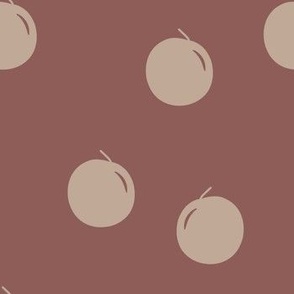This detailed poster-style illustration features a dark brown background, approximately three inches by three inches in size, adorned with light tan or cream-colored circular fruits that resemble cherries. Each of the fruits includes a small, short stem extending from the top. Three complete fruits are centrally positioned, uniformly showcasing a slight dark sliver in the upper right or left corner, which likely represents a gleam or indentation indicating the apple's or cherry's reflective surface. Additionally, two partial semicircles of the fruit appear at the upper right and left corners of the image, adding a sense of depth and framing. The fruits vary slightly in orientation, demonstrating a subtle dynamic arrangement against the brownish-purple hued background.